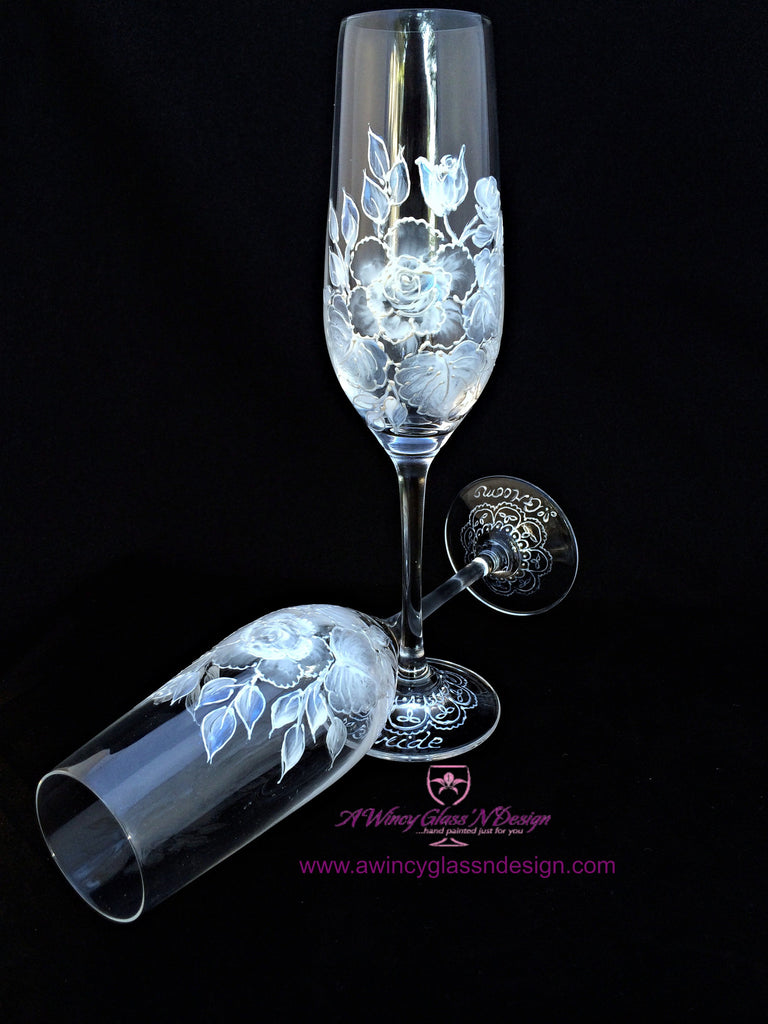Here, we have a color photograph set against a solid black background, showcasing two tall, narrow wine glasses with glass stems and round bases. The glasses feature an intricate design of flowers in white and pale blue hues, accentuated by delicate, light blue petals and ethereal white outlines, lending them an air of fragility and elegance. One glass stands upright, while the other lies toppled on its side with its open end facing left in a diagonal line. Both glasses shimmer softly in the light, highlighting their clear, translucent quality. At the bottom of the image, a pink shield-shaped logo with a wine glass and flower motif, accompanied by the text "E-Wincy Glass and Design, hand-painted just for you," is prominently displayed. Underneath, the website "www.ewincyglassanddesign.com" is written in deep purple, adding a touch of sophistication and tying the composition together. The combination of ornamental carvings at the base and the vibrant floral pattern gives the glasses a distinctive, eye-catching appeal.